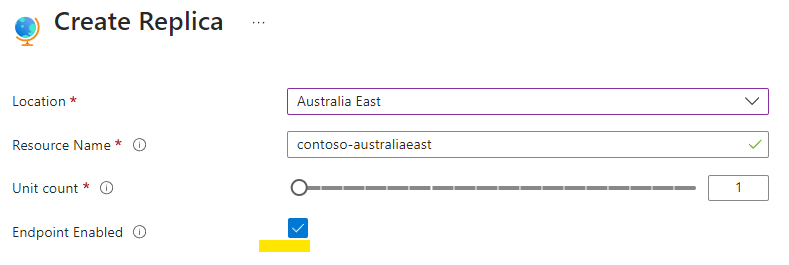The image displays the settings interface of a particular application, focusing on creating a replica. In the top section, the text "Create Replica" is written in black font, accompanied by a globe icon ensconced in a copper harness, reminiscent of a classical globe often seen on a librarian's table. To the immediate right of "Create Replica," there are three gray dots indicating additional settings options.

Moving downwards, there are various form fields, each marked with a red asterisk indicating mandatory fields. The first field is labeled "Location" with a red asterisk. Beneath it is the "Resource Name" field, also marked with a red asterisk and accompanied by a clickable warning button, likely for more information. Similarly, the "Unit Count" field follows the same pattern with a red asterisk and a warning button. The last field in this section is labeled "Endpoint Enabled," again with a warning button beside it.

To the right of these fields, the dropdown selection shows "Australia East," which is currently selected. Below, there is another dropdown showing "Contosa-Australia East," which is also checked. Further down, there's a movable line graph set to the far left, indicating it might be at its minimum value. Below this graph, a blue checkbox is currently checked. Beneath the checkbox, there's a yellow rectangle, and to the right of what appears to be a line dial, the setting is fixed at '1', suggesting the lowest possible setting.

Overall, the interface is rich with details and interactive elements, allowing for precise configuration of the application's replica settings.